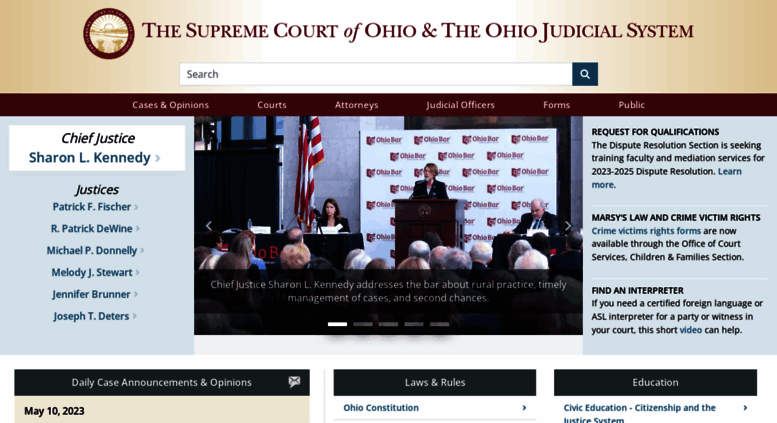This is a detailed caption for the image described:

The homepage of the Supreme Court of Ohio and the Ohio judicial system features an image of a courtroom where Chief Justice Sharon Kennedy is addressing the bar from a podium. She is discussing important topics such as rural practice, timely case management, and providing second chances. The courtroom decor includes an American flag, and two individuals seated at smaller desks on either side of the podium. The audience is visible from behind, listening attentively.

The title "Supreme Court of Ohio and the Ohio Judicial System" is prominently displayed in maroon text. An insignia featuring a maroon circle with yellow images is positioned on the left side of the page. A search bar is available for users, accompanied by navigation links labeled "Cases and Opinions," "Courts," "Attorneys," "Judicial Officers," "Forms," and "Public."

Further information about Chief Justice Sharon Kennedy is noted, including a section listing all the justices. To the right of the primary photograph, additional links are provided for "Request for Qualifications," "Marcy's Law and Crime Victim Rights," and "Find an Interpreter." Below this navigation bar, a greenish-grayish bar contains direct links to "Daily Case Announcements and Opinions" dated May 10, 2023, "Law," "Rules," and "Education." The "Ohio Constitution" is highlighted in blue under the "Law" section, while "Chief Educational Citizenship and the Justice System" is also noted in blue under the "Education" section.